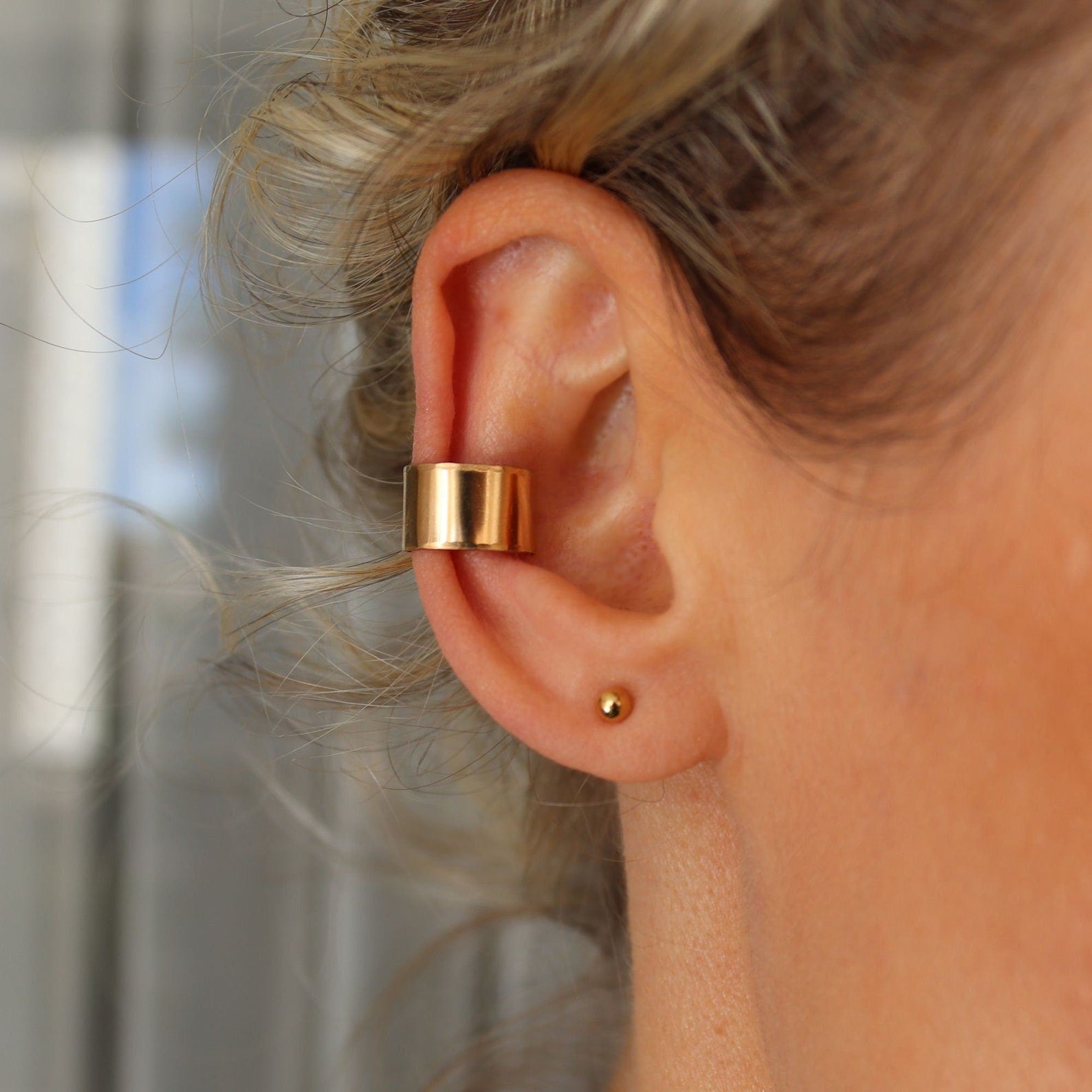This close-up image captures a detailed view of a Caucasian lady's right ear and cheek. The lady's hair, which is a mix of blondish-brown shades with streaks of dark brown and gray, is slightly wavy and is pulled back, with a few wisps escaping behind her ear. On her earlobe, she wears a small gold ball earring. Midway up her ear, a thicker gold cuff earring encircles her conch, standing out against her fair, slightly pink-tinged skin. The background is softly blurred, featuring what appears to be a window with curtains.